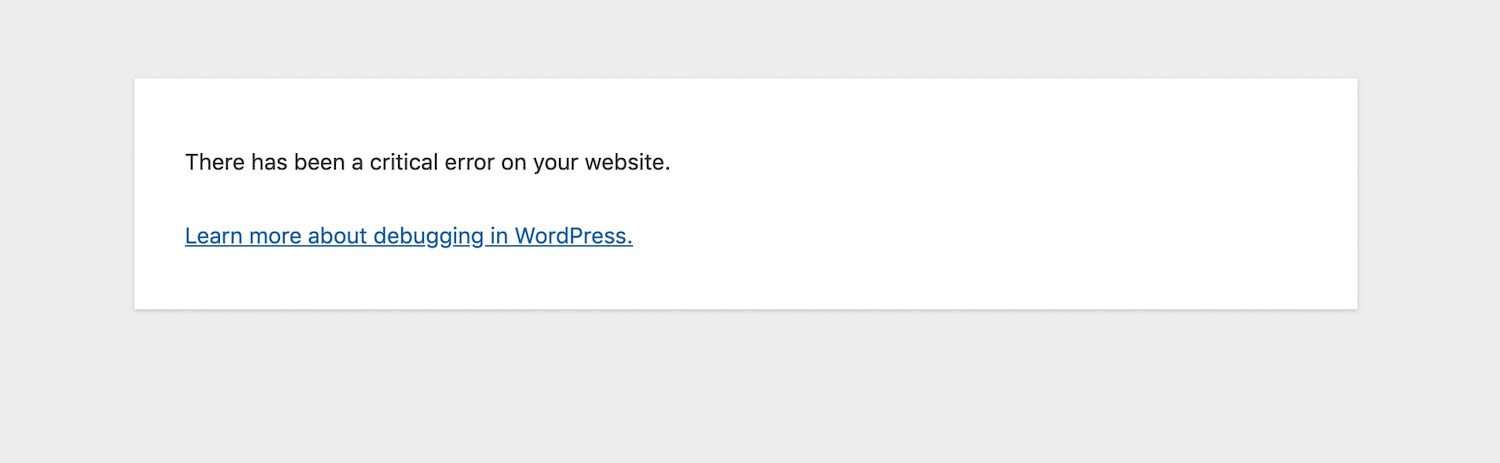This horizontal image appears to be a screenshot or screen grab of a critical error notification that one might see on a smartphone or computer screen. The image has been cropped and zoomed in, focusing on the important message. The background is a medium gray rectangle, thicker at the bottom and sides compared to the top, giving it an asymmetrical look. 

Centered within the gray background is a long, thin white rectangle, bordered by a very thin black line that provides a clear separation from the gray background. Written within the white rectangle in black font is the text: "There has been a critical error on your website." Below this message, in blue font and underlined, the text reads: "Learn more about debugging in WordPress."